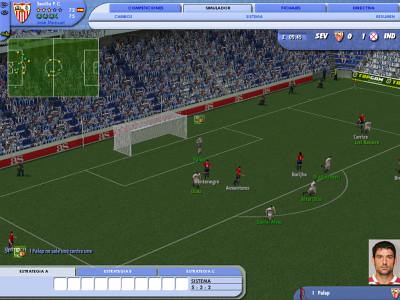A nostalgic screenshot from an early-era soccer video game, capturing the essence of classic sports gaming. The image presents a green soccer field marked with white boundary lines. Scattered across the field are players in distinct uniforms: some clad in red, others in blue, and a few in white. Under each player is a name tag, color-coded in white or green. Dominating the left side of the field is a large goal. In the background, stands filled with fans dressed in blue and white create a lively atmosphere. At the top of the screenshot, a mini-map overview of the field displays player positions and ongoing action. Additionally, game statistics are prominently displayed, offering the player quick insights into the match dynamics.